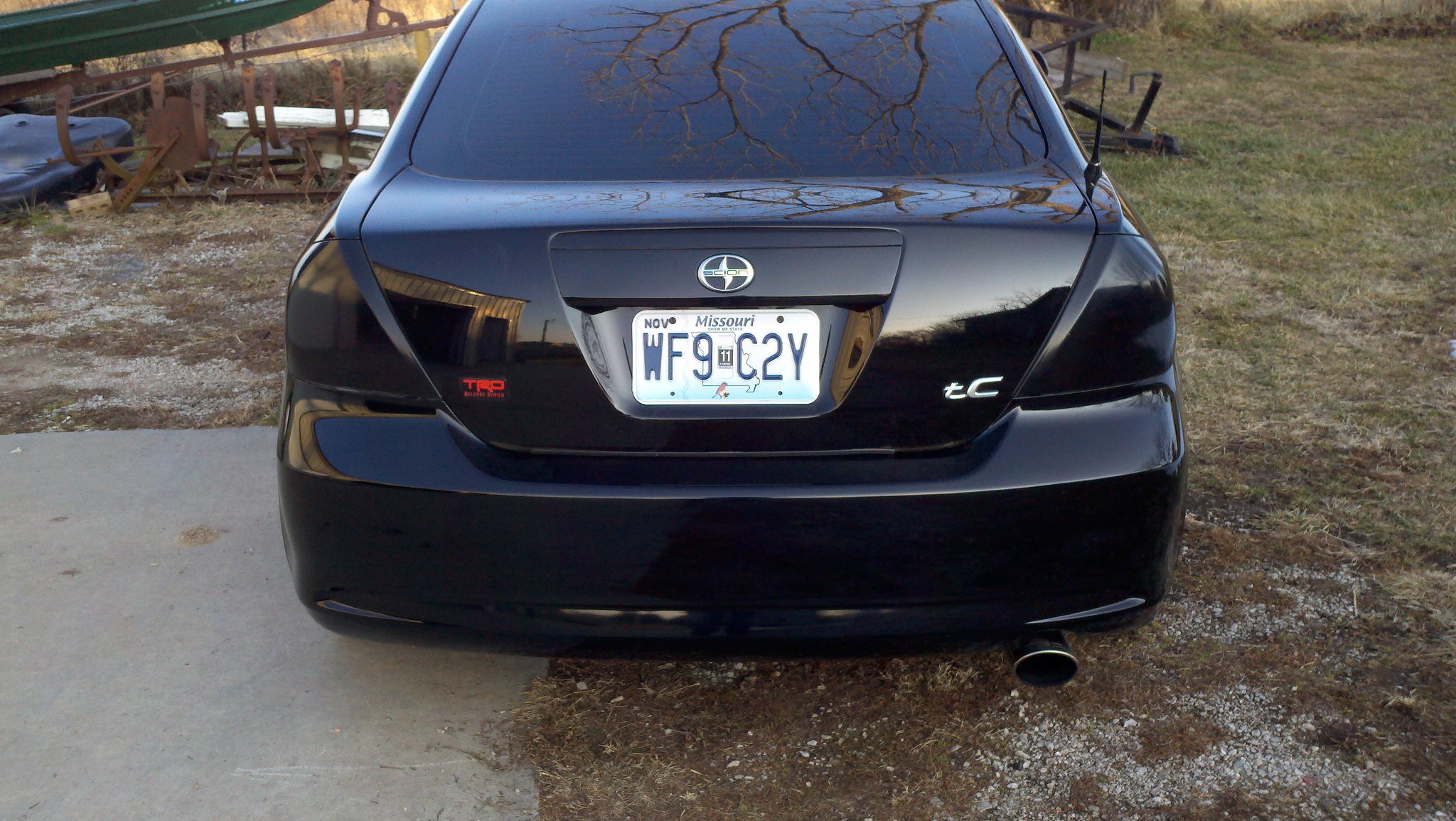In this detailed photograph, we see the rear of a black Skyon sedan parked in a muddy and grassy field. It's evident that the location is quite possibly a rural area, potentially a farm with some property. The Skyon has undergone several modifications: its brake lights have been blacked out, and the windows are heavily tinted, contributing to its sleek all-black appearance. The license plate is from Missouri, displaying the number WF9C2Y. This faint turquoise and white plate stands out starkly against the dark backdrop of the car. Additional notable details include a silver logo centered on the trunk and a red decal whose text is not readable. There's also a lowercase "tC" branding on the bottom right of the trunk. Surrounding the car, you can discern cut green grass, a concrete pad, scattered debris including something blue and wooden, and a decrepit green boat on a rusted trailer. The photograph seems to be taken from an angle that captures both the car and its immediate, somewhat cluttered surroundings.